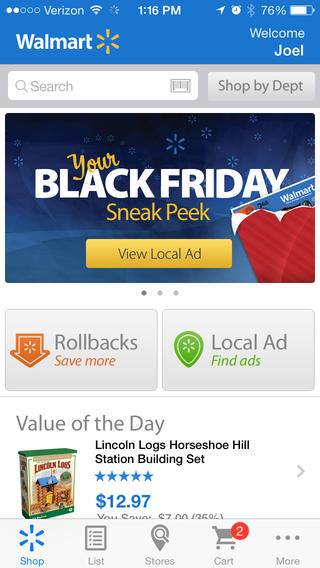The image displays the Walmart website as viewed on a mobile device. In the top left corner, the status bar indicates the device is connected to Verizon with Wi-Fi enabled. A loading symbol resembling radiating lines in a circular shape is present. The signal strength indicator shows two out of five bars filled. The time is 1:16 PM, displayed in small white bolded font. Adjacent to this is an upward diagonal arrow, indicating location services are active, followed by an alarm clock icon showing the alarm is set. The Bluetooth symbol is next, and towards the far right, a battery icon is displayed with the number "76%" indicating the battery charge level.

Below this status bar, the prominent Walmart logo is visible. The header has a light gray background with a blue Walmart banner that reads "Welcome Joel" in white lettering, with Joel in bold. To the right of the search bar, there's a button labeled "shop by DEPT" for departments.

A Black Friday banner is prominently featured below this. The banner initially says "your" in a playful, curly, slanted yellow font. Following this, in large, bold, white capital letters, it says "BLACK FRIDAY." Below this, in a traditional circular yellow Walmart font, it reads "sneak peek." In the right corner of the banner, an illustration shows a present opening to reveal a Walmart flyer inside.